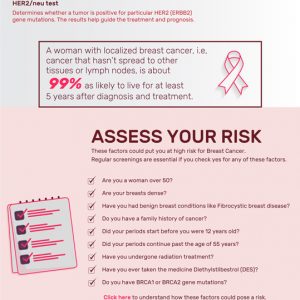The image depicts a detailed infographic related to breast cancer diagnostics and prognosis. At the top, it mentions the results of new tests determining whether a tumor is HER2-positive. HER2-positive tumors are associated with a specific type of breast cancer. The infographic highlights a woman diagnosed with localized breast cancer, meaning the cancer hasn't spread to other tissues or lymph nodes.

Statistics indicate that this woman has a 99% likelihood of living for at least five years following her diagnosis and treatment. The number "99%" is prominently displayed in pink, while the remaining text is in a dark purple color. Additionally, there’s a prominent pink breast cancer awareness ribbon symbol.

The infographic includes a section titled "Assess Your Risk," accompanied by a checklist. All the checkboxes to the left of the listed risk factors are checked, emphasizing the thoroughness of the risk assessment provided by the infographic.